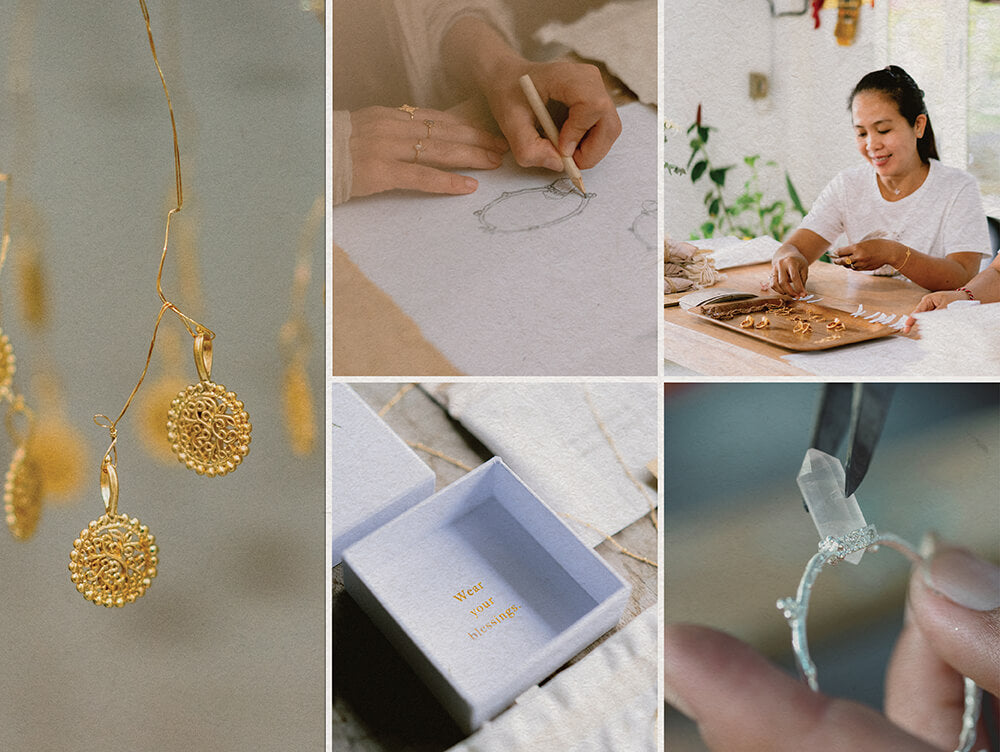The image is a detailed collage of five panels depicting various aspects of jewelry making and presentation. The far-left panel features a close-up of two golden pendants adorned with beaded edges, hanging intricately from teardrop connectors on what resembles a branch. Moving to the center panel, the top square captures a hand sketching a bracelet design on white paper with a beige pencil, the artist's fingers adorned with three rings. Below it, there is a white box inscribed with "Wear your blessings," likely a jewelry box with a paper insert typically found in packaging. The top-right square shows a woman with long dark hair in a white shirt inspecting or arranging items on a copper tray, in a room with white walls and plants in the background, hinting at an arts and crafts setting. Lastly, the bottom-right panel shows a close-up of a pair of tweezers carefully inserting a long gem into a silver bracelet, portraying a step in the jewelry crafting process. This composition altogether appears to be an elaborate advertisement showcasing various stages and elements of jewelry creation and packaging.